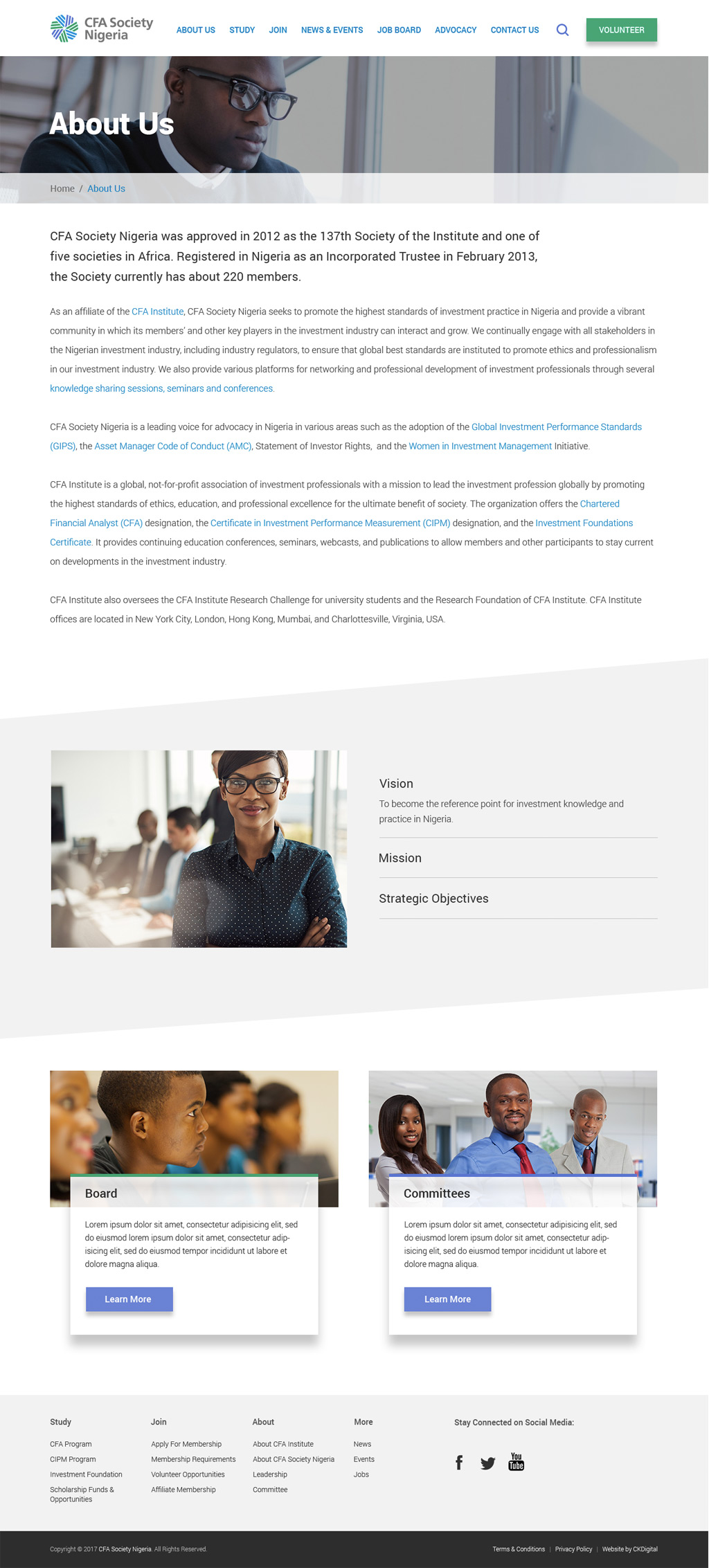The image depicts the CFA Society Nigeria, showcasing various elements of their mission and activities. 

At the top, a CT scan image symbolizes balance, study, and enjoyment in using the lens of professional development. This includes sections for a job board, advocacy initiatives, contact information, a magnifying glass symbolizing scrutiny, and volunteer opportunities highlighted in green. 

In the central part of the image, a man is depicted wearing reflective glasses, and he is positioned in front of a laptop, although the laptop screen appears blank. This represents the professionals engaged in the industry and the introspective nature of their work.

The caption highlights the "Great Minds" home session, emphasizing the dedication of the society to intellectual growth. The CFA Society Nigeria was approved as a society in 2012 by the Institute and officially registered in Nigeria as an incorporated trustee in February 2015. The society boasts around 220 members.

As an affiliate of the CFA Institute, the CFA Society Nigeria strives to uphold the highest standards in professional practice and training within a supportive environment where members can interact and grow. The society actively engages with all stakeholders in Nigeria, advocating for industry interests and setting a standard for professional development.

Additionally, there is a section dedicated to the society's vision and committee structures, reflecting the operational intensity and commitment to fostering professional excellence in Nigeria.